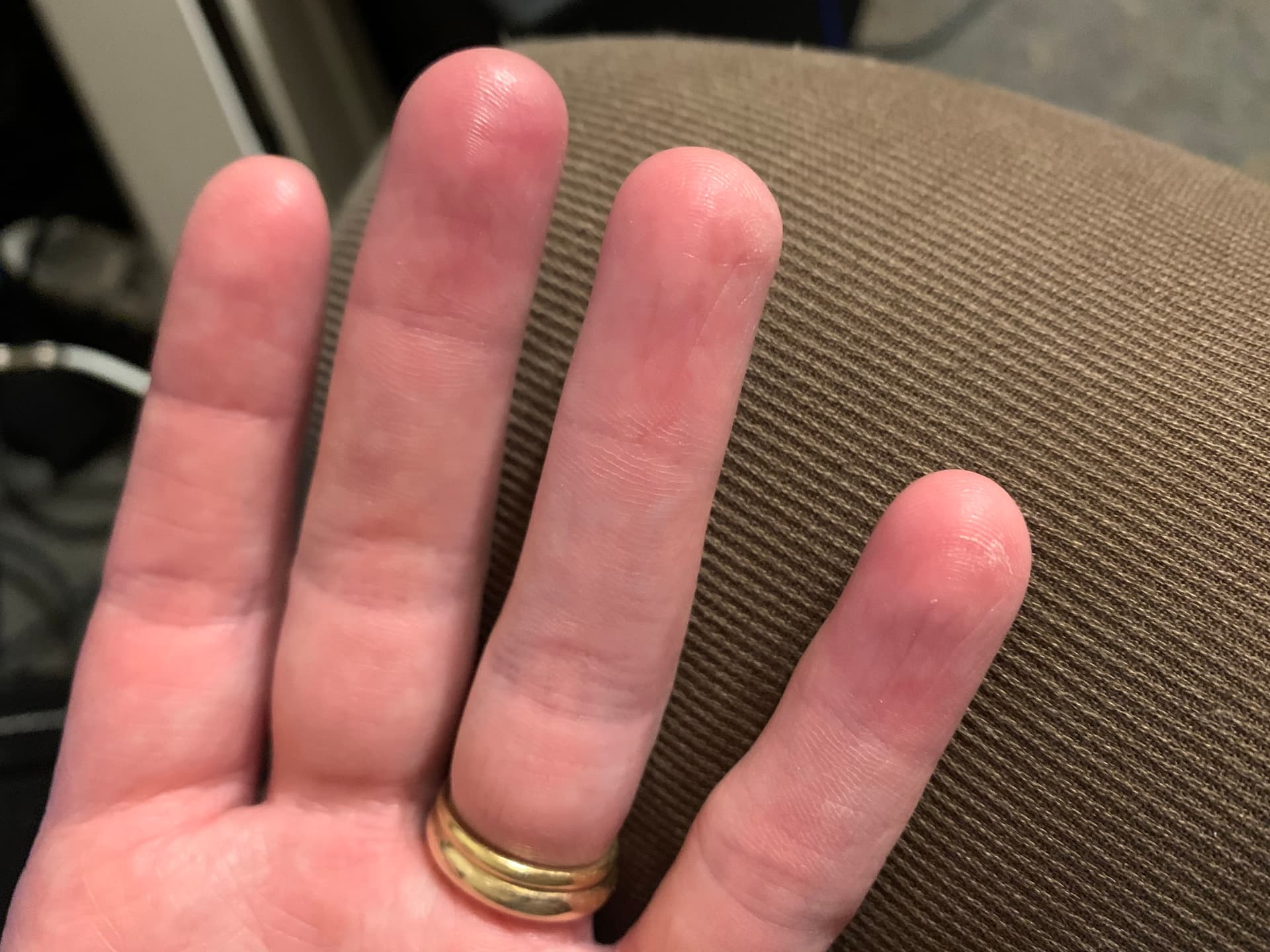This detailed photograph captures a close-up of the left hand of a person, palm side up, with four visible fingers—the thumb is not visible. The hand appears to be that of a Caucasian individual, possibly male, and features plump, rough fingers with a pink and white coloration. Adorning the ring finger is a large gold wedding band. The hand is gently resting on the arm of a brown couch with horizontal stitching. In the blurred background, several unidentifiable household items are present, including a silver rectangular object that could be an air-conditioning unit, suggesting the scene is set within a home.